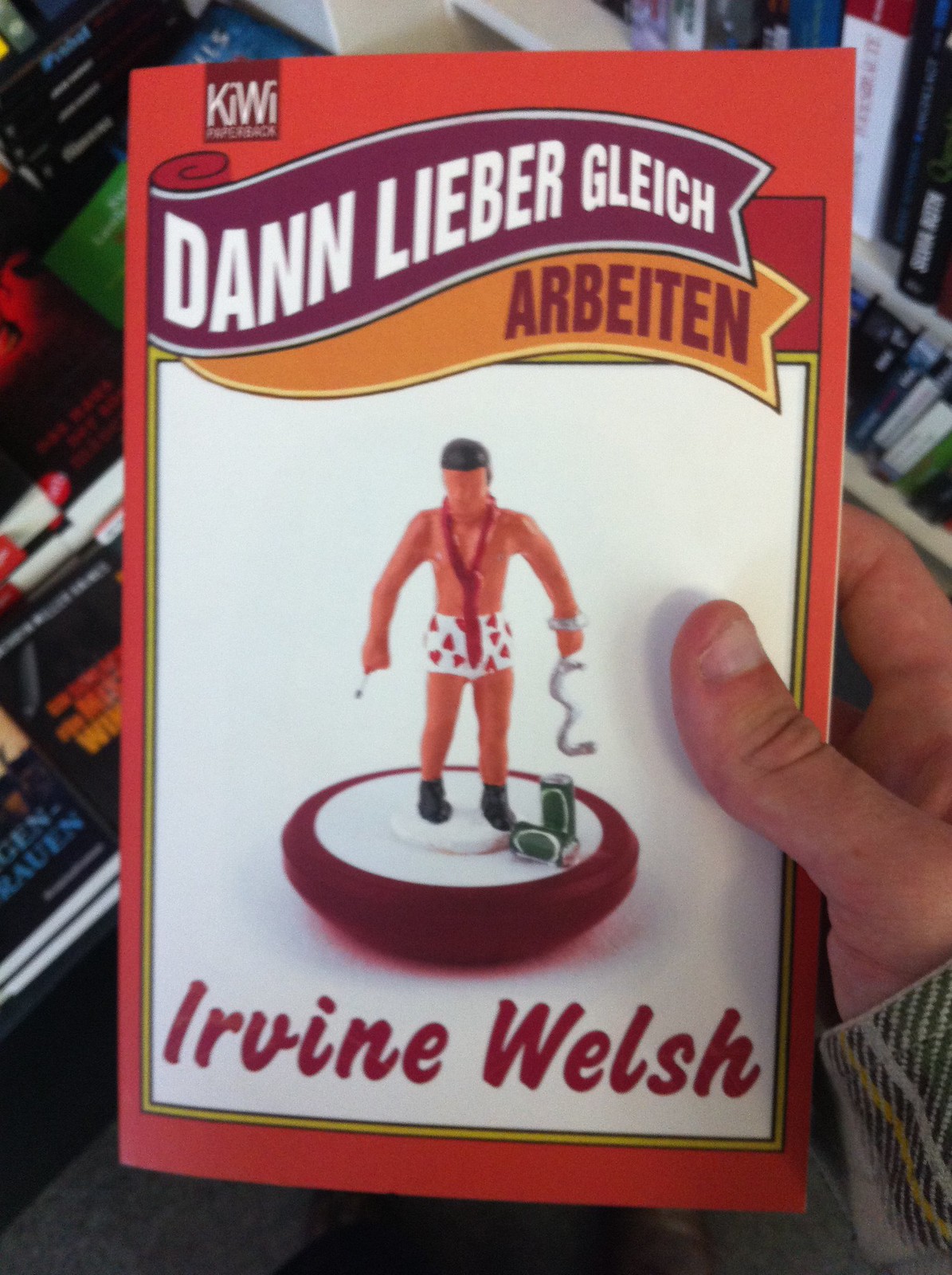The slightly out-of-focus photograph captures a hand holding what appears to be a German paperback book, identifiable by the text "Kiwi Paperback" at the top. The book's cover prominently features the names "Don Lieber Glietsch" and "Ivern Welsh," suggesting confusion over the authors or perhaps multiple contributors. The title seems to be "R. Bertin," though there is also mention of an "Arbeiten," indicating content related to work. The central image on the cover depicts a male doll standing on a platform, wearing white shorts with red hearts, a red tie, and dark shoes or boots. He is accessorized with an open shackle on one wrist and holds a key or similar object in one hand, and possibly a cigarette and beer cans, hinting at a playful or satirical nature. The book is held in front of a cluttered background featuring a box of pencils, crayons, other small utensils, and a stack of books, which adds to the scene's chaotic and colorful atmosphere.